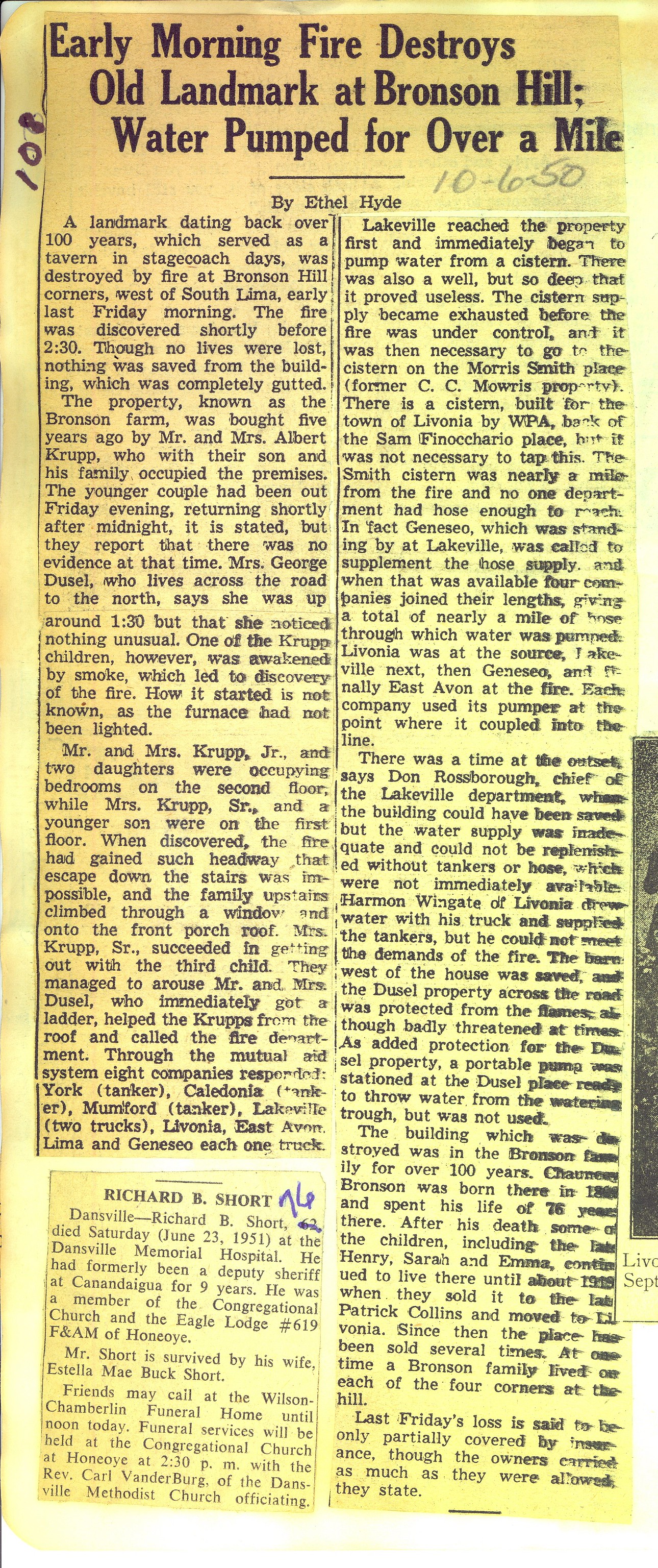This is an image of a very old, worn-out newspaper clipping that appears to have been xeroxed. The paper, once white, has now turned a yellow, brownish color due to fading over time. The article is long and rectangular, with the text arranged in two substantial columns separated by a thin line. The font used is black Times New Roman, typical of standard newsprint.

The headline of the article reads, "Early Morning Fire Destroys Old Landmark at Bronson Hill, Water Pumped for Over a Mile." Just below the headline, the date "10-6-1950" (October 6, 1950) is written in pencil. The article is credited to Ethel Hyde. The content of the article spans multiple paragraphs and delves into the details of the fire and the landmark that was destroyed. To the left of the clipping, there are additional markings made with a marker.

Overall, this is an evocative and nostalgic piece that captures a moment in history, detailing the destruction of a significant landmark by fire.